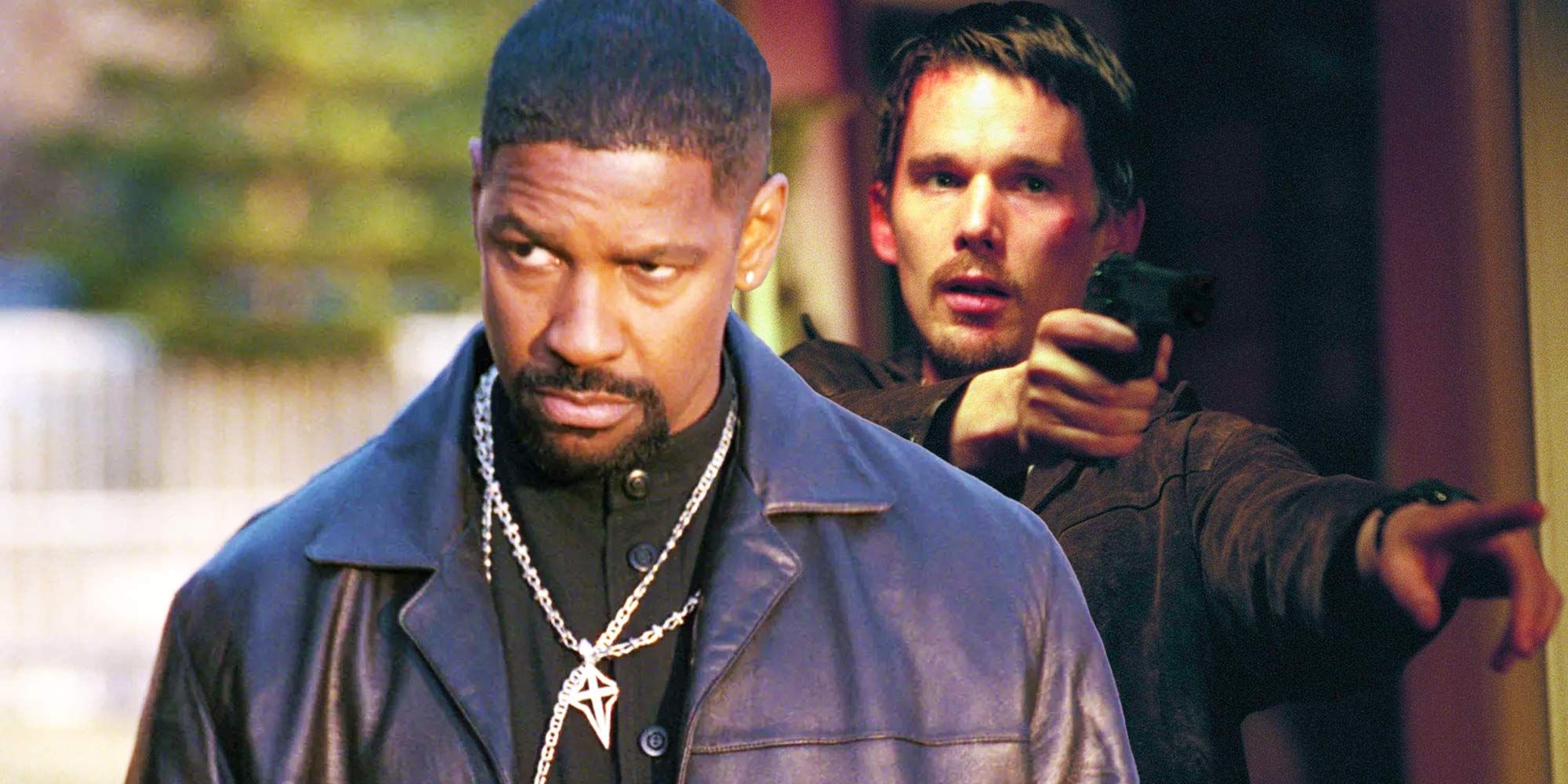In the promotional collage of the movie "Training Day," on the left side, Denzel Washington, an African American male with a very short buzz cut hairstyle, stands with a serious expression. He wears a black shirt under a black leather jacket, adorned with silver chain necklaces. His character exudes a commanding presence, with broad shoulders and a contemplative gaze directed slightly downward to the left. Behind him, the blurred background features green trees indicative of an outdoor setting.

On the right side, we see Ethan Hawke, a Caucasian male with short brown hair, captured from mid-chest up. He dons a dark button-up shirt and is intensely focused, his mouth slightly open, suggesting alarm or urgency. In his right hand, he firmly grips a black Beretta handgun, pointed towards the right side of the image. His left hand is extended forward with his index finger pointing, enhancing the tension in the scene. The background on this side is darker, possibly depicting an indoor setting with contrasting light. This composite image encapsulates the high-stakes, gritty atmosphere of "Training Day," which premiered in the early 2000s.